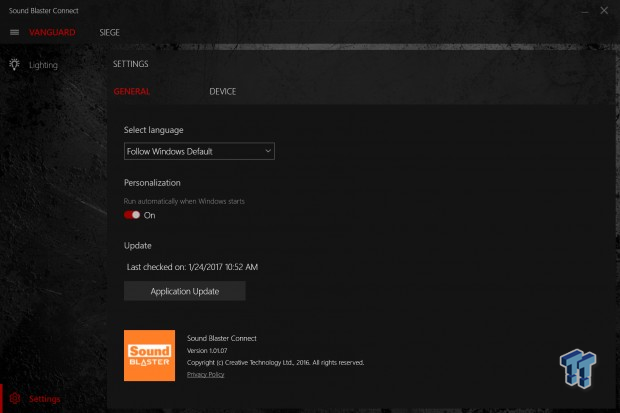The image appears to be a screenshot from a website featuring the Sound Blaster Connect application. The overall background of the interface is black, enhancing the visibility of various UI elements. In the top left corner, the text "Sound Blaster Connect" is prominently displayed, while an 'X' button is situated to the right, likely for closing the application.

On the left side of the image, there is some red text, but it is indistinguishable due to the blurriness. Below this text, the word "Lighting" is visible.

Further down, there is a section with multiple selectable options, including "Settings," "General," and "Device." The interface also allows the user to select a language through a dropdown menu labeled "Select Language." 

Additionally, there is a feature for personalization, which is currently turned on. Another section titled "Update" indicates that the last check for updates was performed on January 12, 2017, at 10:52 am. Below this, there is an "Application Update" option.

At the bottom right corner of the image, the letters "Ts" are visible.